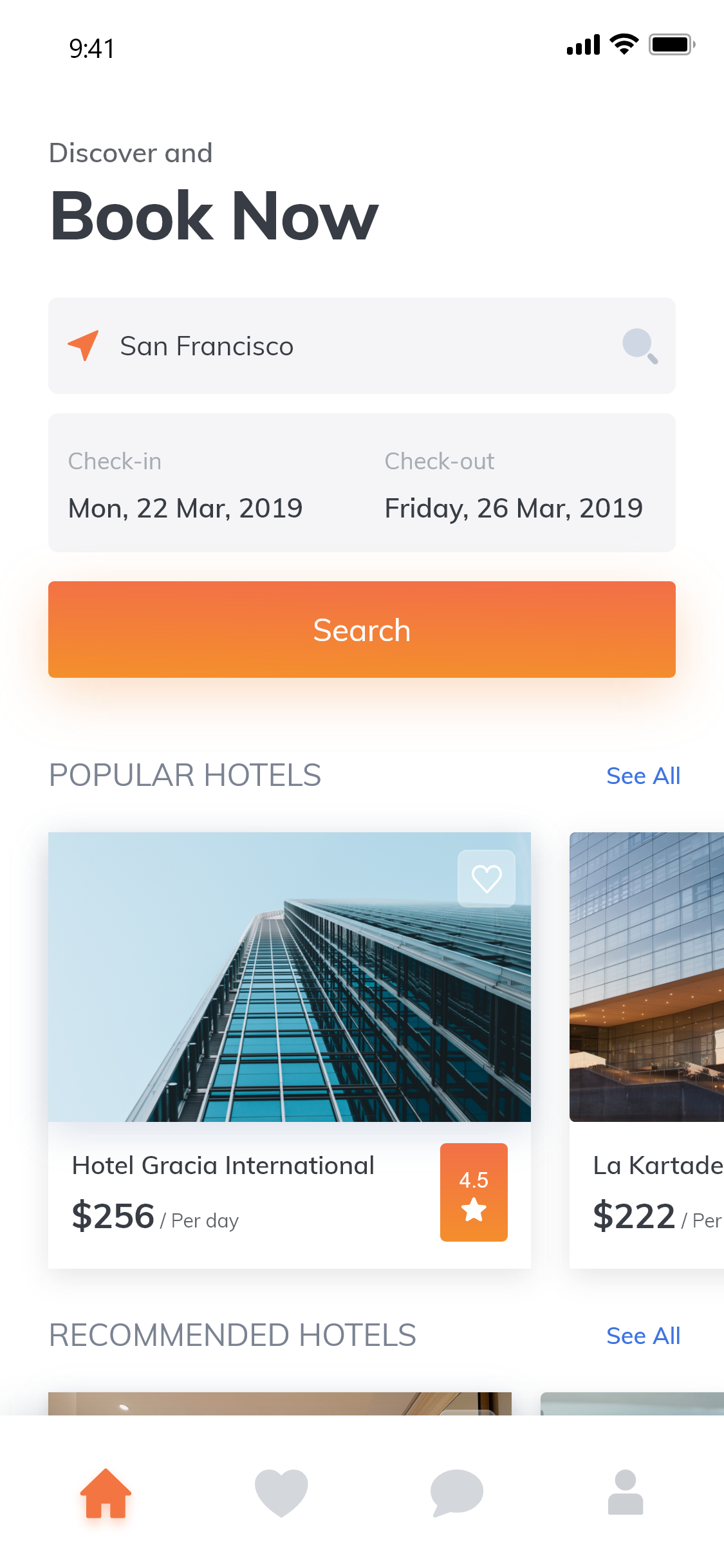Screenshot Description of a Hotel Booking Website:

The screenshot captures a hotel booking website displayed on a smartphone, with the phone's status bar indicating it is 9:41 AM, showing full network connectivity with four bars, a complete Wi-Fi signal, and a fully charged battery icon. 

At the top of the website interface, there is a header with the phrase "Discover and Book Now," where "Discover and" is in small grey font, while "Book Now" is prominently displayed in a larger black font. Below this header, an orange pointer arrow icon is positioned next to the text "San Francisco," and a search button featuring a magnifying glass icon is situated on the right.

Further down, a section for checking in and checking out is displayed in grey text, with the specific dates shown in black: check-in on Monday, March 22, 2019, and check-out on Friday, March 26, 2019. A large orange search button is located beneath this section.

Following the search button, the page displays the heading "Popular Hotels" along with a "See All" button, indicating that users can scroll sideways and possibly downwards to view more options. Visible thumbnails show the various hotels listed, including partial views of hotels to the right that are cut off mid-image.

The first thumbnail presents the exterior view of a building with a glass facade against the sky, labeled "Hotel Gracia International" at a rate of $256 per day, complemented by a four and a half star rating. To the right, partially visible, is another hotel named "La Cartada," priced at $223 per day, though the thumbnail cuts off some of the details.

Below this section, another category titled "Recommended Hotels" follows a similar thumbnail layout, displaying a grid of hotel options with visible cut-offs to indicate more hidden content.

At the bottom of the screen, there are navigation buttons for the home, favorites (heart), messages (speech), and profile, with the home button highlighted in orange, signifying it is the currently selected option.